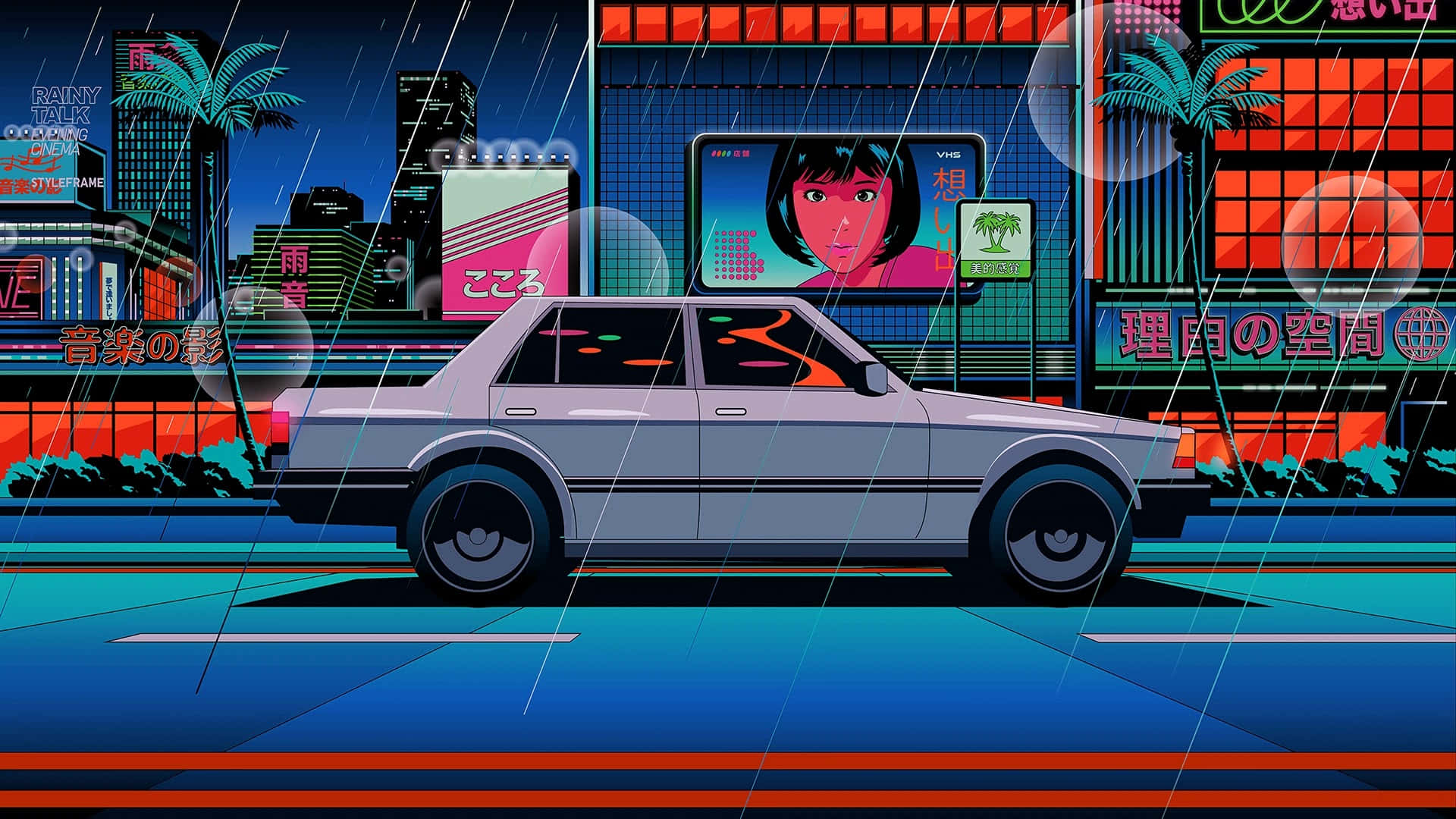This is a stylized screenshot from an anime cartoon movie set in Japan, depicting a rainy night scene. The primary focus is on a gray, old-fashioned four-door compact sedan with black rims, black side stripes, and visible partial side views of the taillights and headlights. The car is driving down a strikingly blue city street with red divider lines and occasional white markings. The backdrop features vibrantly colored buildings with red windows and non-English neon signs, possibly Japanese writing. One prominent advertisement displays a young Japanese girl with short, shiny black hair reaching her shoulders, exuding a bright pink and purple hue. Additionally, there's a gray logo in the upper left corner that appears to say "rainy talk." Palm trees are positioned alongside the sidewalk, lending a hint of tropical ambiance amidst the urban environment punctuated by skyscrapers and diverse architectural forms. Raindrops streak across the scene, intensifying the atmospheric depiction of a classic city progressing through a vibrant, rainy night.